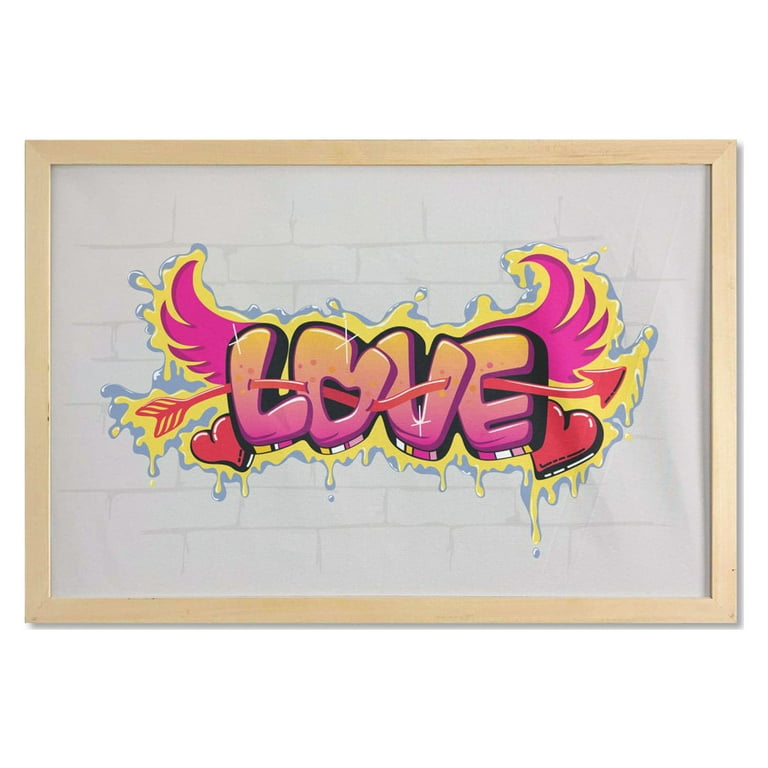This framed artwork is rendered in a digital painting style, featuring the word "LOVE" prominently. The letters are bold block shapes, shaded from pink and orange at the bottom to yellow at the top, with a subtle dripping paint effect. A distinctive, curved red arrow winds sinuously through the letters, adding a dynamic element to the composition. On either side of "LOVE," there are two hearts, and behind the word are two upturned pink wings accentuating the design. The entire piece is set against a backdrop of a light gray brick wall, designed with vague black brick-like etchings for texture. Twinkle stars add a whimsical touch within the letters. The artwork is bordered by a light wooden frame that complements its vibrant yet urban aesthetic.